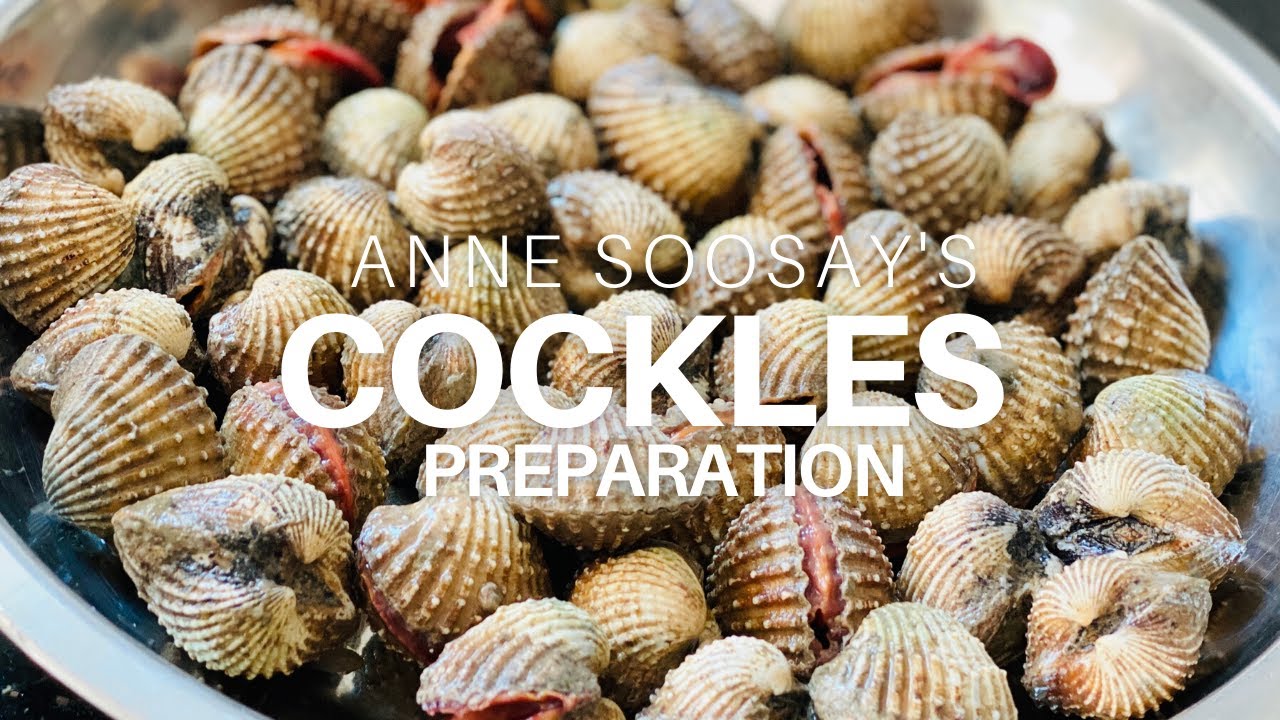This is an image of what appears to be the front page of a cookbook. Featured prominently in the center of the page is a rectangular photograph showcasing a shallow, stainless steel bowl filled with an assortment of cockles. The cockles, nestled snugly in the bowl, exhibit a tapestry of colors and textures—ranging from light browns and darker browns to hints of black, various shades of red, and touches of olive green. Each cockle is distinctly in its closed position, adding to the visual appeal and sense of freshness in the image. Overlaying the photograph, in elegantly contrasting white font, is the title: "Anne Sosa's Cockles Preparation," providing an inviting introduction to the culinary delights within.